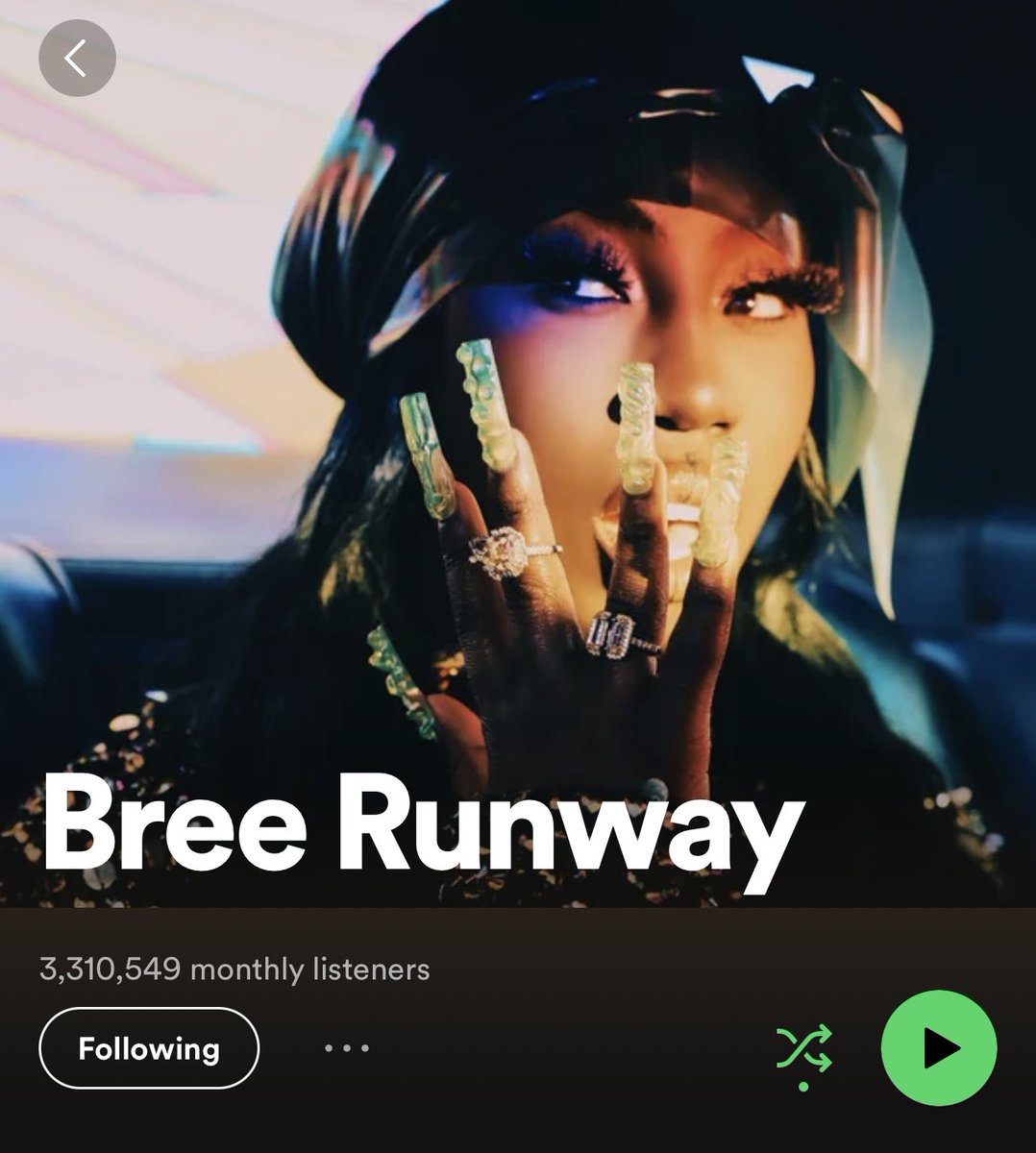This digital image features an African American woman who exudes the presence of a singer, and likely is Bree Runway, given the textual context within the image. She has striking, very long and thick eyelashes that draw attention to her eyes, which are looking out from the corners. Draped over her head is a fashionable scarf, adding an element of style to her overall look. The image appears to be digitally enhanced, suggesting some photoshopping has been done to perfect the visual.

Adorning her fingers are multiple rings, including a large, prominent diamond ring on her middle finger. Her artificial nails are notably long and feature a textured design with small bubble-like details. Her mouth is slightly open, revealing a set of impeccably white and straight teeth. She is positioned inside a car.

Additionally, the image includes a title at the bottom, "Bree Runway," along with a statistic indicating "3,310,549 monthly listeners." Accompanying buttons for following (a green and black arrow), options (three dots), and other interactive features are also present, suggesting this might be a capture from a music streaming platform.